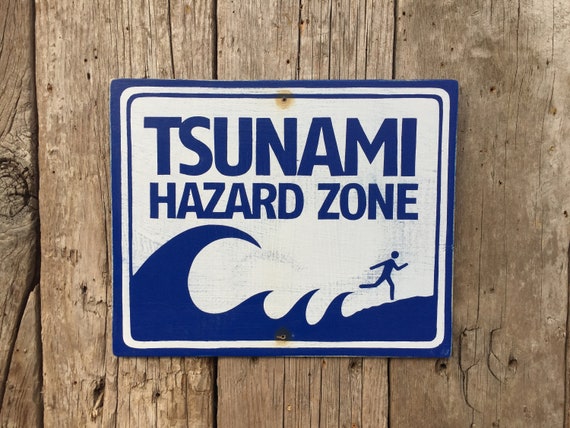The photograph features a weathered, dark blue and white "Tsunami Hazard Zone" sign nailed to a set of distressed wooden panels, likely part of a fence or an old wooden building. Positioned centrally within the image, the sign displays large, navy blue text that reads "Tsunami Hazard Zone" against a white background. Beneath the text, an illustration depicts a series of waves, with a particularly large one representing a tsunami, and a small stick figure man running away towards the right, indicative of fleeing the shore. The sign's dark blue border separates it neatly from the aged, weather-beaten wood, which has clearly suffered from years of exposure to saltwater, suggesting a coastal location. Rust rings around the two nails securing the sign further emphasize its age and prolonged exposure to the elements.